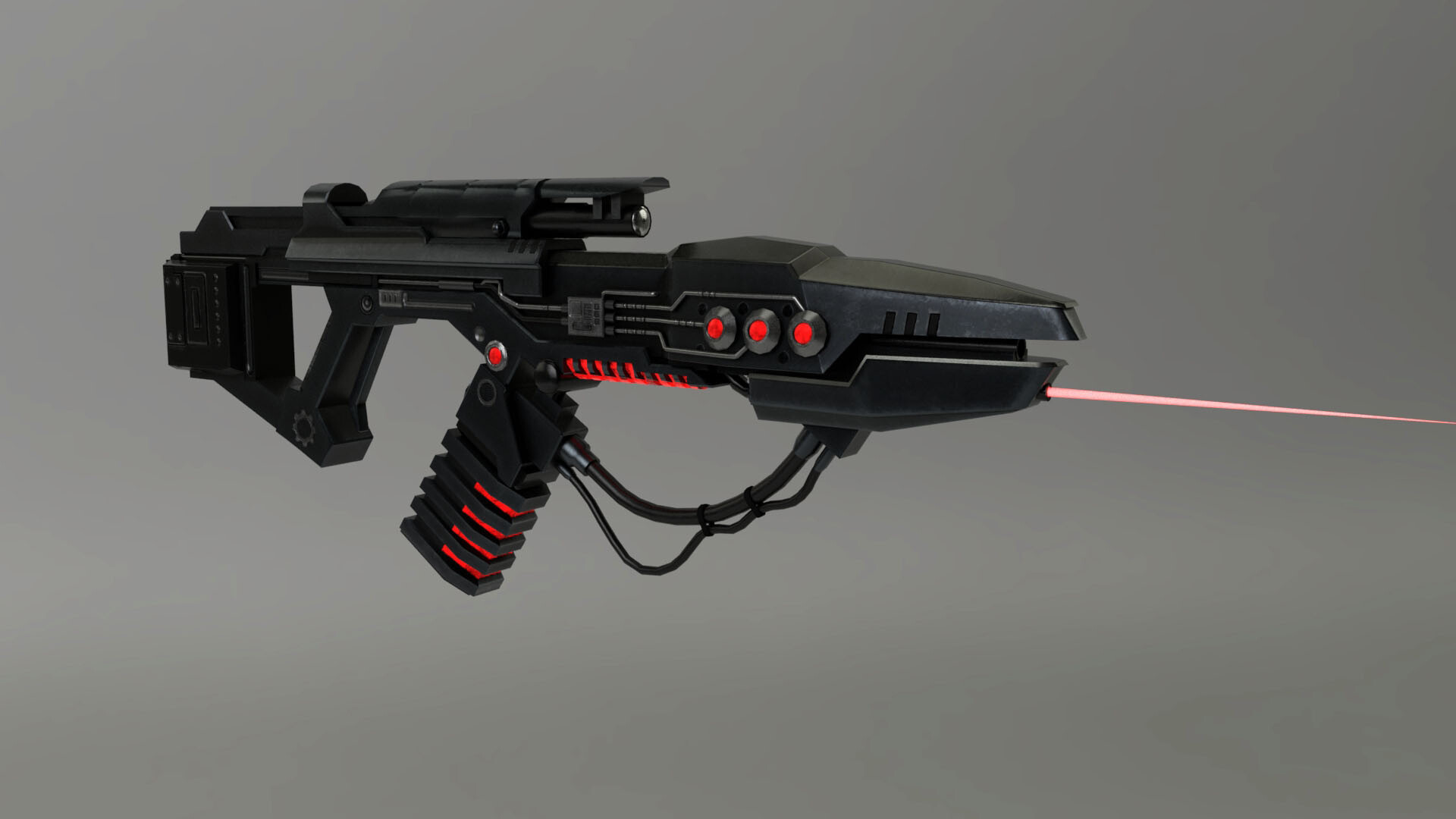The image depicts a large, black laser gun with intricate details and several illuminated red lights. The gun, which is held like a handgun, features a substantial handle at the back and a sleek, black body. Prominently, it emits a thin, pinkish-red laser beam from its front. The weapon's design includes a scope positioned on top for aiming, and the front barrel displays three circular red lights. Additional red lights are observed on the handle and under the gun's belly. The color red also appears on a cartridge and a button on the side of the ammo clip. The backdrop of the image is predominantly dark gray with lighter gray shading, complementing the striking appearance of the futuristic laser weapon.